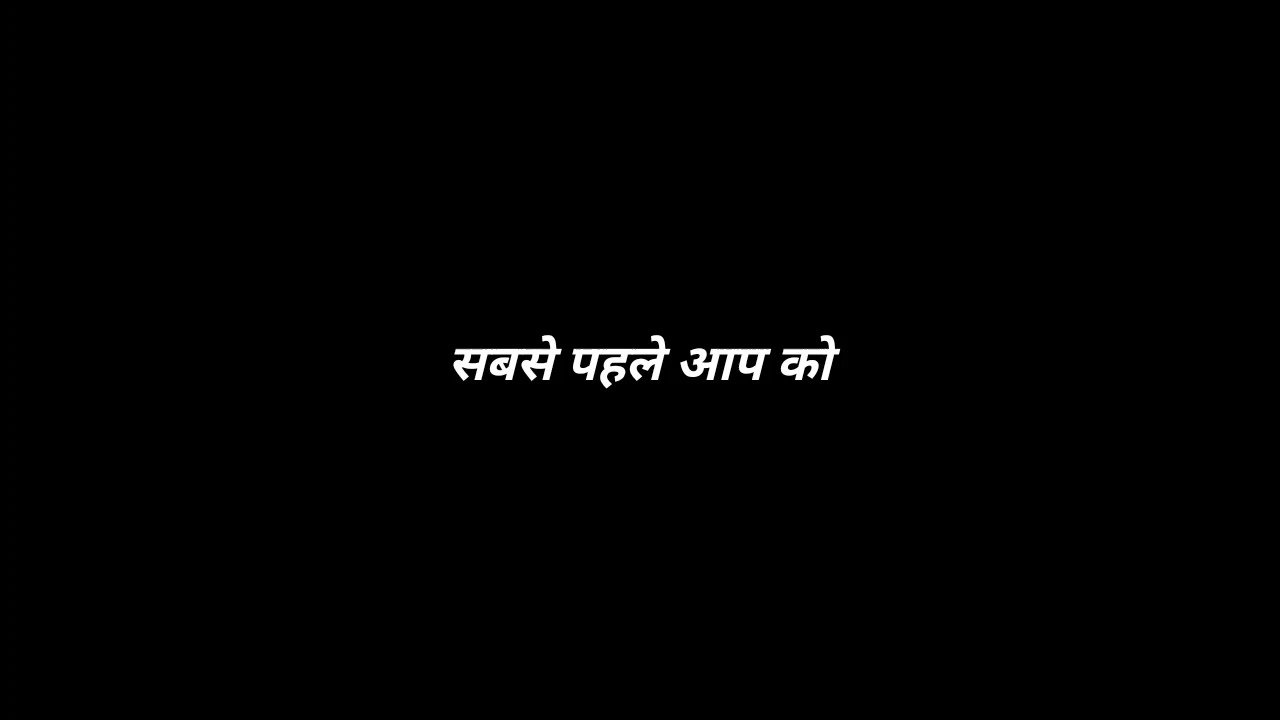In the image, a horizontal and rectangular frame with a completely matte black background showcases a single line of text centrally. The text consists of four distinct words written in a bright white, foreign script that resembles Sanskrit or a Middle Eastern language. Each word is separated by a small, thin horizontal bar positioned above them. The first word appears to contain three characters, where the first and last characters look identical, and the middle one resembles an 'A.' The following words are also made up of characters that resemble Latin letters but are distinctly foreign. The simple layout and stark contrast between the black background and the white text make for a striking, minimalist visual.